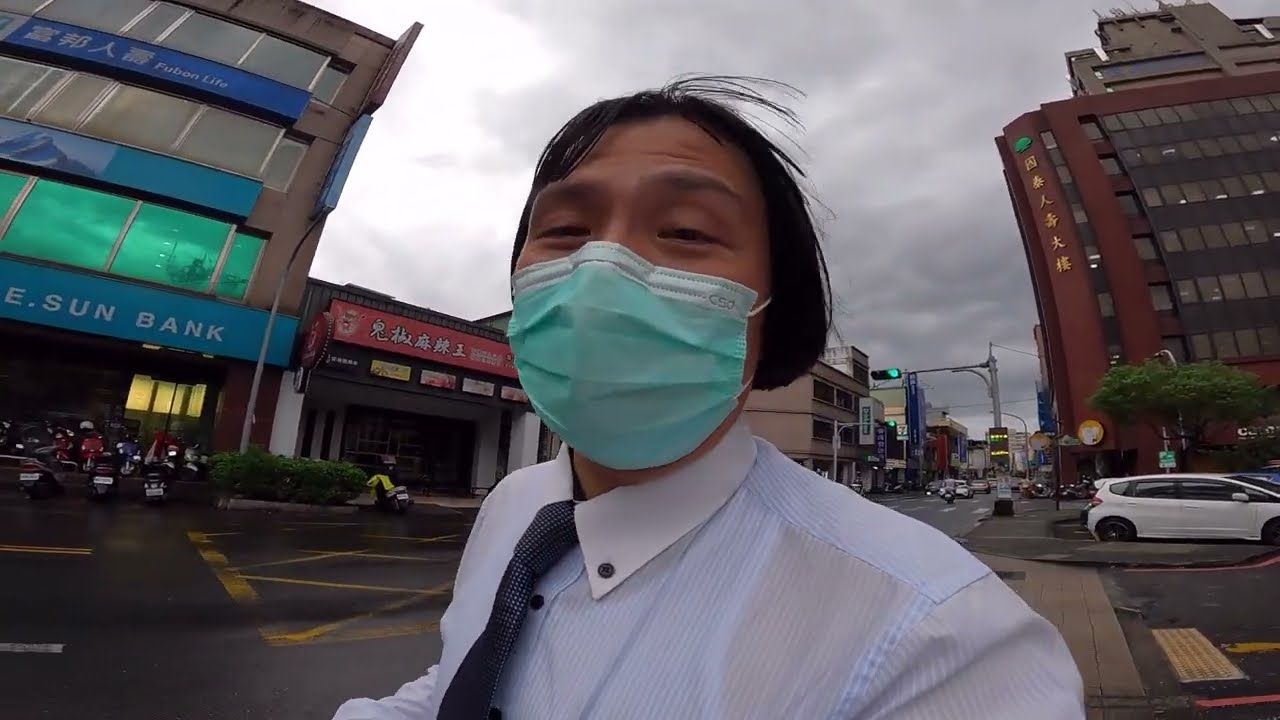The image captures a horizontally aligned rectangular close-up of a man, who looks like a doctor, wearing a white button-down shirt with a button-down collar, adorned with a subtle vertical stripe pattern, and a black tie with a small gray checkered pattern. His short black hair and dark eyes are partially concealed by an aqua-colored surgical mask. He stands in an urban environment, possibly in an Asian country, inferred from the presence of buildings with Asian script and symbols in the background. The cloudy sky overhead casts a gray hue across the scene. 

The man is positioned in front of a crosswalk on one side of a street, with a bustling downtown area behind him. Buildings in the backdrop appear slightly warped, leaning left and right reminiscent of a funhouse effect. One notable building across the street has an awning that reads partially as "Sunbank," alongside another building marked "Fubon Life." A prominent red building features vertically aligned yellow symbols. Additionally, green traffic lights and several cars, including a white SUV parked on the lower right-hand side, populate the road. Motorcycles can be seen parked near the Sunbank sign, adding to the dynamic urban scenery. Overall, the composition highlights the juxtaposition of the man's poised appearance against the lively and somewhat distorted cityscape, enriched with a mix of architectural elements and cultural markers.